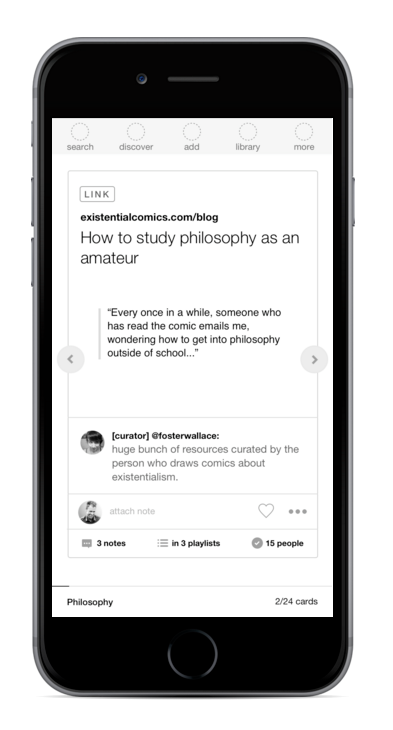The image showcases a black smartphone screen displaying a web page. At the top, there is a white navigation bar featuring icons and text labels. From left to right, the labels read: "Search," "Discover," "Add," "Library," and "More," each represented by corresponding circular icons.

Beneath the navigation bar, a white box with a gray border contains a link, "takesintentionalcomics.com/blog," followed by the text, "How to study philosophy as an amateur." Below this, a swipe left and right button frame the text, "Every once in a while, someone who has read the comic emails me wondering how to get into philosophy outside of school."

Further down, a gray horizontal line separates the content from additional information which reads, "A huge bunch of resources created by the person who draws comic about existentialism." At the bottom of the screen, a profile picture is visible accompanied by a heart icon. This detailed depiction encapsulates the visual elements and content displayed on the smartphone screen.